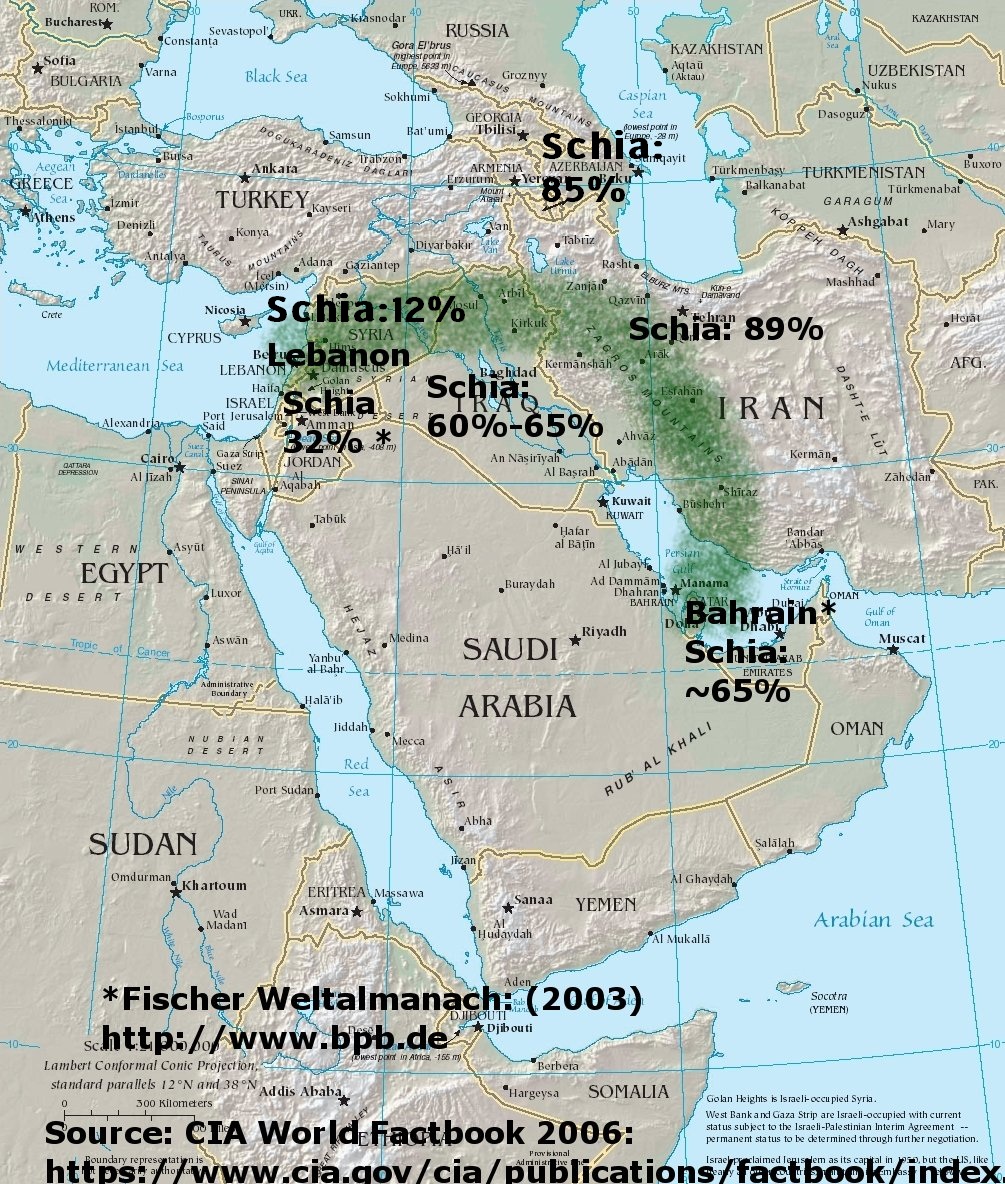This image is a detailed map of the Middle East, extending from Southeast Europe to the edge of Central Asia, specifically Uzbekistan. In the top left corner, the map includes Bulgaria, while the top right corner reaches the borders of Uzbekistan. The central focus of this map is on Saudi Arabia and its neighboring countries.

A prominent feature of the map is the green spray paint-like highlights over several regions, particularly the left portion of Iran, extending through Syria, the northern half of Iraq, and parts of the Levant. The map also includes five key labels indicating the Shia Muslim populations in various countries. Near Turkey, a label notes the Shia population at 85%. Over Iran, the Shia population is indicated to be 89%. In Syria, the Shia population is marked at 12%, in Lebanon at 32%, and in Iraq, it ranges from 60% to 65%. Additionally, the Shia population in the Bahrain area is roughly 65%.

At the bottom of the map, there is black text providing sources and references, namely "Fischer Weltalmanach 2003" accessible through "http://bpd.de" and data from the "CAA Factbook 2006" with another reference to the "CAA Factbook" website.